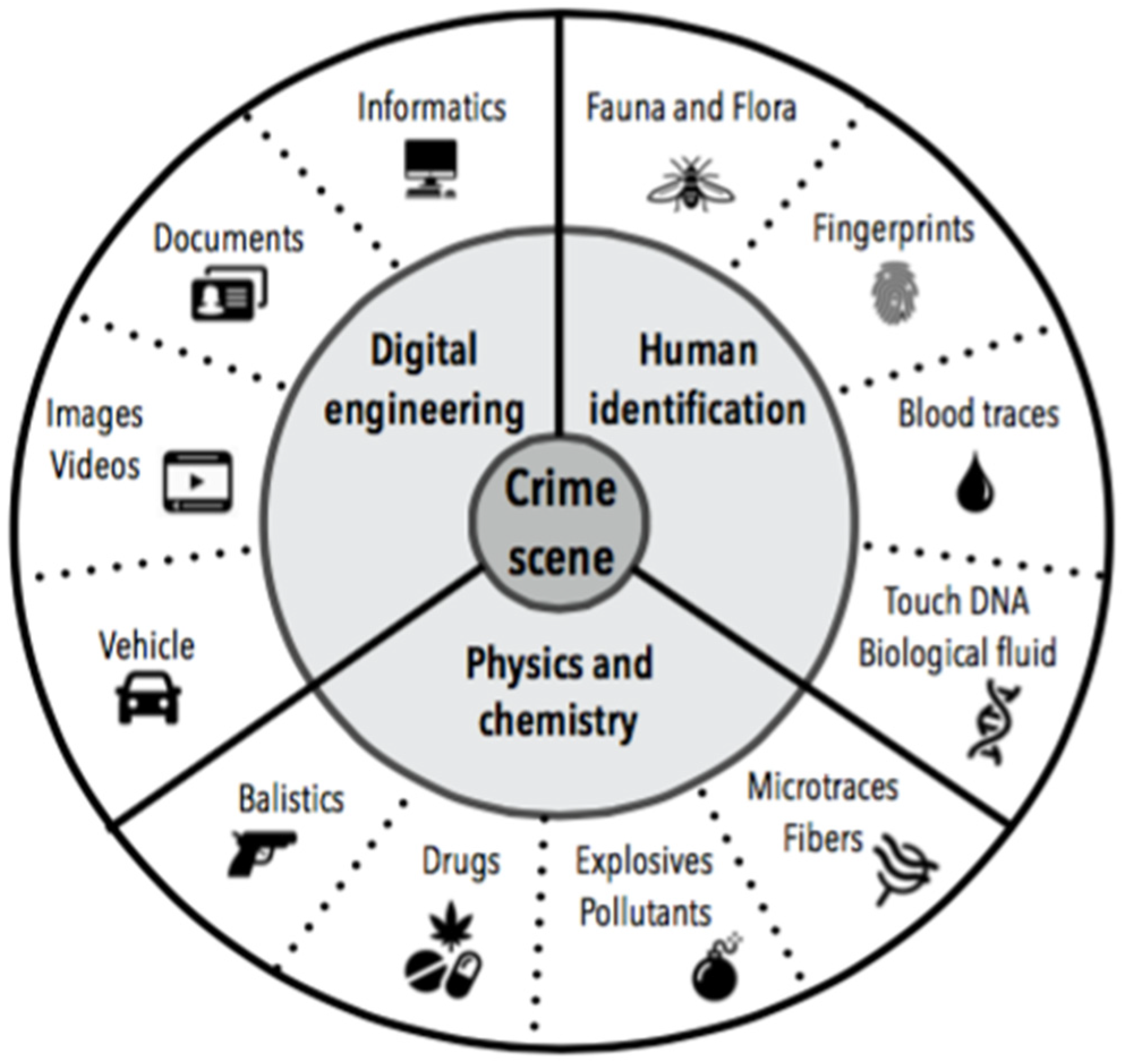The image is a detailed black-and-white circular diagram set against a white background. At the center of the diagram is a small white circle labeled "Crime Scene" in black text. Radiating outward, the diagram features concentric circles divided into sections with text and small illustrations that categorize different elements of forensic investigation.

The innermost circle beyond the central "Crime Scene" label is partitioned into three sections, labeled "Digital Engineering," "Human Identification," and "Physics and Chemistry," arranged clockwise starting from the top left. Each of these categories is then further divided into detailed subcategories. 

For "Digital Engineering," the subcategories include informatics, documents, images, videos, and vehicle, each accompanied by relevant illustrations such as a computer monitor, an ID card, and a car. 

"Human Identification" encompasses subcategories like fingerprints, blood traces, touch DNA, and biological fluid, illustrated by images of a fingerprint, blood droplets, and a DNA strand.

"Physics and Chemistry" is divided into microtraces, fibers, explosives, pollutants, drugs, and ballistics, with each section featuring corresponding illustrations such as a microscope for microtraces, a bomb for explosives, and a gun for ballistics.

The outermost ring of the diagram is defined by a solid black border and is segmented with dotted lines radiating from the center. The diagram visually explains the different layers and components involved in crime scene investigation, providing a comprehensive overview of the forensic processes and categories, each with related illustrations to enhance understanding.